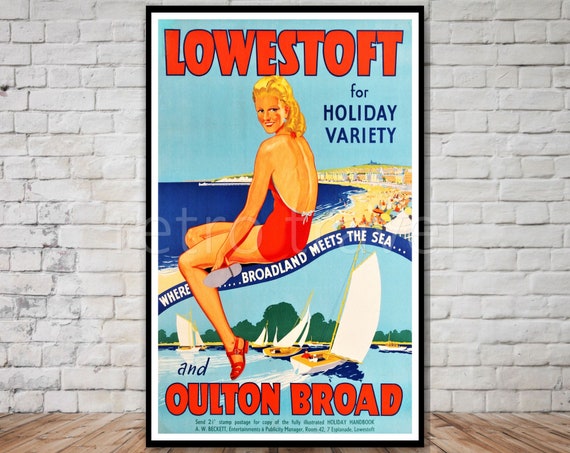The image is a vintage advertisement poster from the 1950s for holiday vacations in Lowestoft, leaning against a white brick wall on a wooden floor. The poster, framed in black, features a vibrant illustration of a woman in a one-piece bathing suit, gazing to the right with a beach scene in the background. The banner reads "Lowestoft for Holiday Variety Where Broadland Meets the Sea" in large red letters, set against a light blue background. A serene seaside ambiance is depicted with waves lapping on the shore, sailboats dotting the water, and a bustling beach crowd. The detailed illustration uses colors like dark blue, light blue, green, red, tan, beige, and black. Towards the bottom, a fine print invites viewers to send a 21-cent stamp for a fully illustrated holiday handbook from A.W. Beckett, the entertainments and publicity manager, highlighting immersive holiday experiences in Oulton Broad.